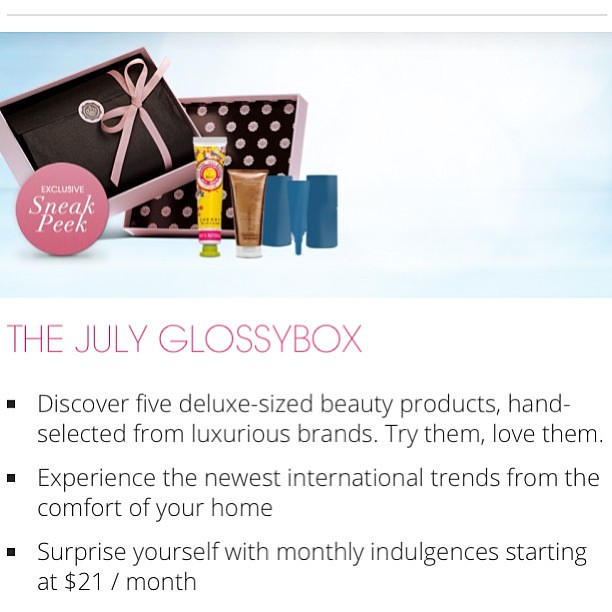The image depicts an advertisement for the July Glossy Box, a makeup box subscription service. At the top of the ad, there is an image of the subscription box against a light blue background, with a bright white area in the center, creating an effect as if the sun is shining on it. The box itself is predominantly pink with a big pink ribbon and contains black lining with pink polka dots. The open box reveals various beauty products, including tubes of lotion and other skincare items, with packaging in colors such as yellow, pink, green, gold, and blue. Some items seem to be organized in what might be a makeup bag tied with a pink ribbon, with a clasp designed in a round emblem.

In front of the box, a pink circular badge displays the words "Exclusive Sneak Peek" in white letters. Below the image, the text reads, "The July Glossy Box" in all capital purple-pink font. Further down are three bullet points in black font highlighting the subscription's main features: 

1. Discover five deluxe size beauty products, hand-selected from luxurious brands.
2. Try them, love them, and experience the newest international trends from the comfort of your home.
3. Surprise yourself with monthly indulgences starting at $21 per month.